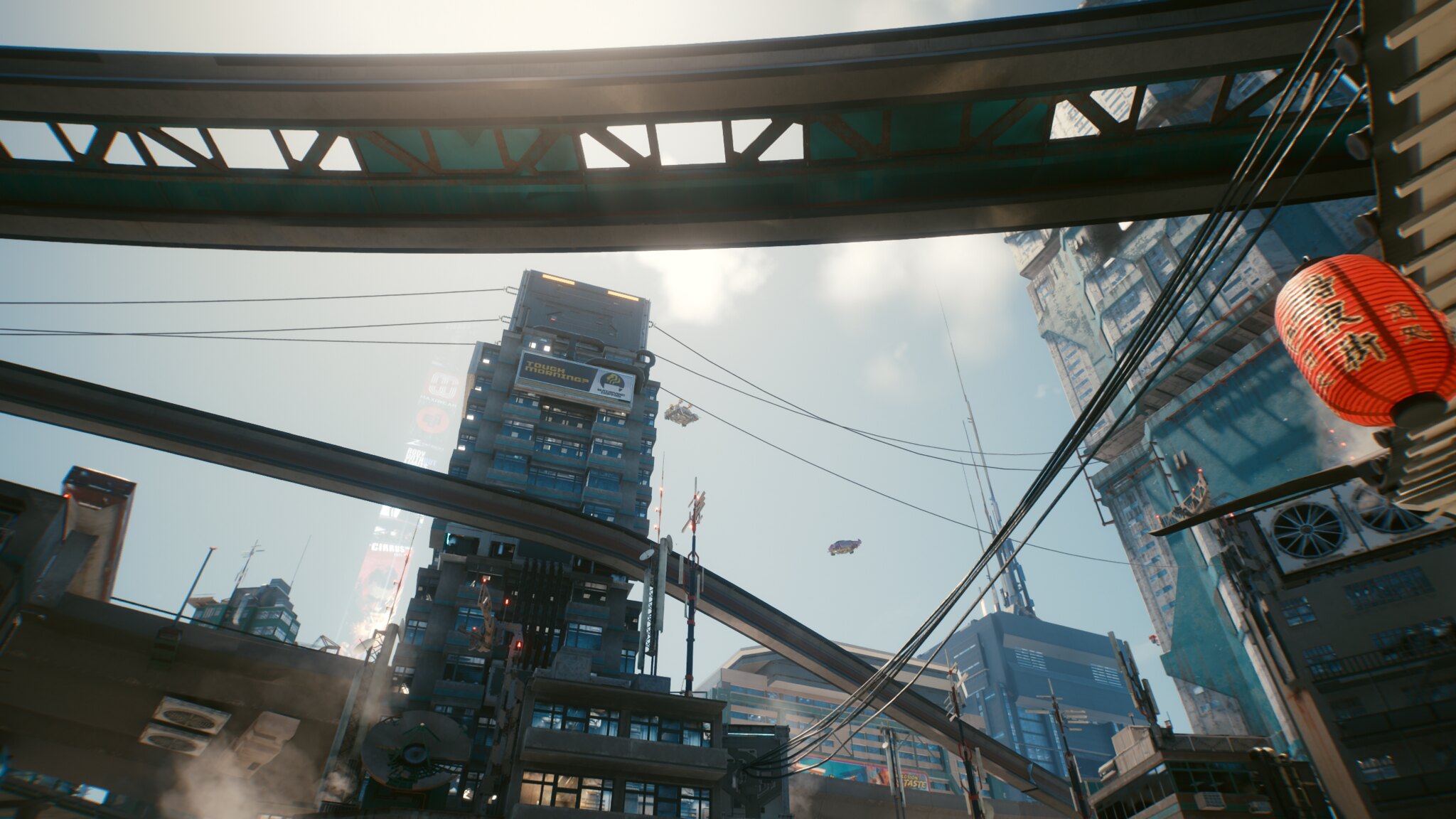The image is a ground-up perspective capturing an urban cable car system. Vibrant, balloon-shaped cars are suspended by cables, traversing in opposite directions between a towering structure that resembles a parking garage. The mid-ground features a Chinese restaurant, identifiable by a red lantern adorned with Asian script and a fan on the building's exterior. Rooftops pepper the scene, overlooked by a prominent building with a large antenna. A distinctive brown railroad bridge or elevated structure, perforated with square cut-outs, extends horizontally across the frame. Smaller buildings with glass windows dot the area, while a wisp of smoke ascends in the background. On the left, additional larger buildings complete this bustling cityscape.